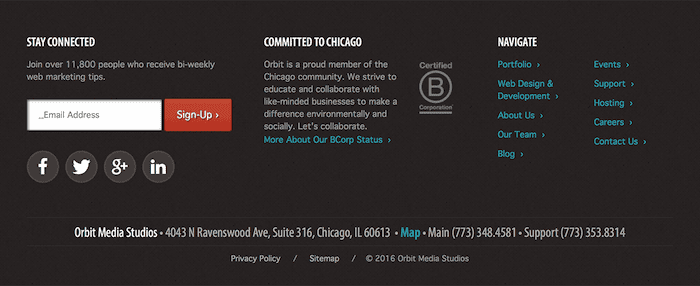The image features a large black box with the header "Stay Connected" displayed prominently in white text. Below this headline, there is an invitation for viewers to join a community of over 11,800 people who receive bi-weekly web marketing tips. An email address input box is provided, followed by a prominent red "Sign Up" button with a right arrow.

Beneath the sign-up section, there are circular icons representing Facebook, Twitter, and Gmail. To the right of these icons is a message outlining the company’s commitment to the Chicago community. It states: "Orbit is a proud member of the Chicago community. We strive to educate and collaborate with like-minded businesses to make a difference environmentally and socially. Let's collaborate."

Highlighted in blue text is a link, "More about our B Corp status," accompanied by a right arrow. Adjacent to this, there is a B Corporation certification logo and the word "certified" is displayed within a circle.

Further to the right, under the heading "Navigate" in white text, there are several navigation options listed in blue, each with a right arrow next to them: Portfolio, Web design and development, About us, Our team, Blog, Events, Support, Hosting, Careers, and Contact us.

Finally, at the bottom of the box, Orbit Media Studios' contact details are listed:

- Address: 4043 North Ravenswood Avenue, Suite 316, Chicago, Illinois 60613
- Phone: Main 773-348-4581
- Support: 773-353-8314

Additionally, links to the Privacy Policy and Site Map are provided alongside the indication that the information is © 2016 by Orbit Media Studios.